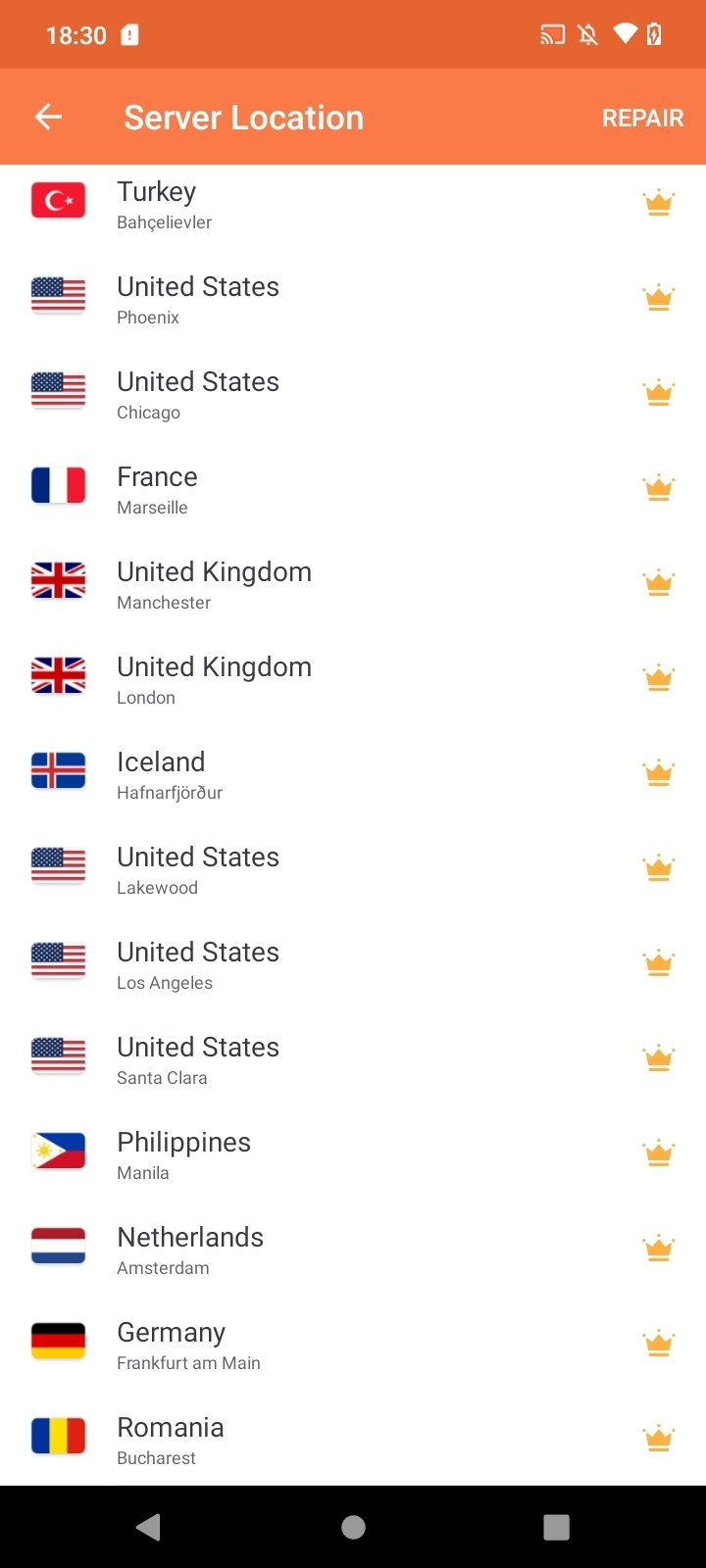This image is a smartphone screenshot captured at 18:30, featuring various interface elements and specific server location details. In the top-right corner, there are several icons: the first resembles a screen with a Wi-Fi signal, followed by a mute sound icon, another Wi-Fi icon, and a battery indicator. Below this section, the header has an orange border transitioning to a lighter shade of orange, with a left-facing arrow labeled "Server Location" and a "Repair" button.

The main content area lists locations vertically, each marked by their corresponding national flags and names. The locations include:

1. Turkey
2. Baja, Bolivia
3. United States - Phoenix
4. United States - Chicago
5. France - Marseille
6. United Kingdom - Manchester
7. United Kingdom - London
8. Iceland - Hafnafjordur
9. United States - Lakewood
10. United States - Los Angeles
11. United States - Santa Clara
12. Philippines - Manila
13. Netherlands - Amsterdam
14. Germany - Frankfurt am Main
15. Romania - Bucharest

The bottom border is black, embedding a left-facing arrow, a Home button, and a Stop button. This detailed description captures the structure and content of the screenshot comprehensively.